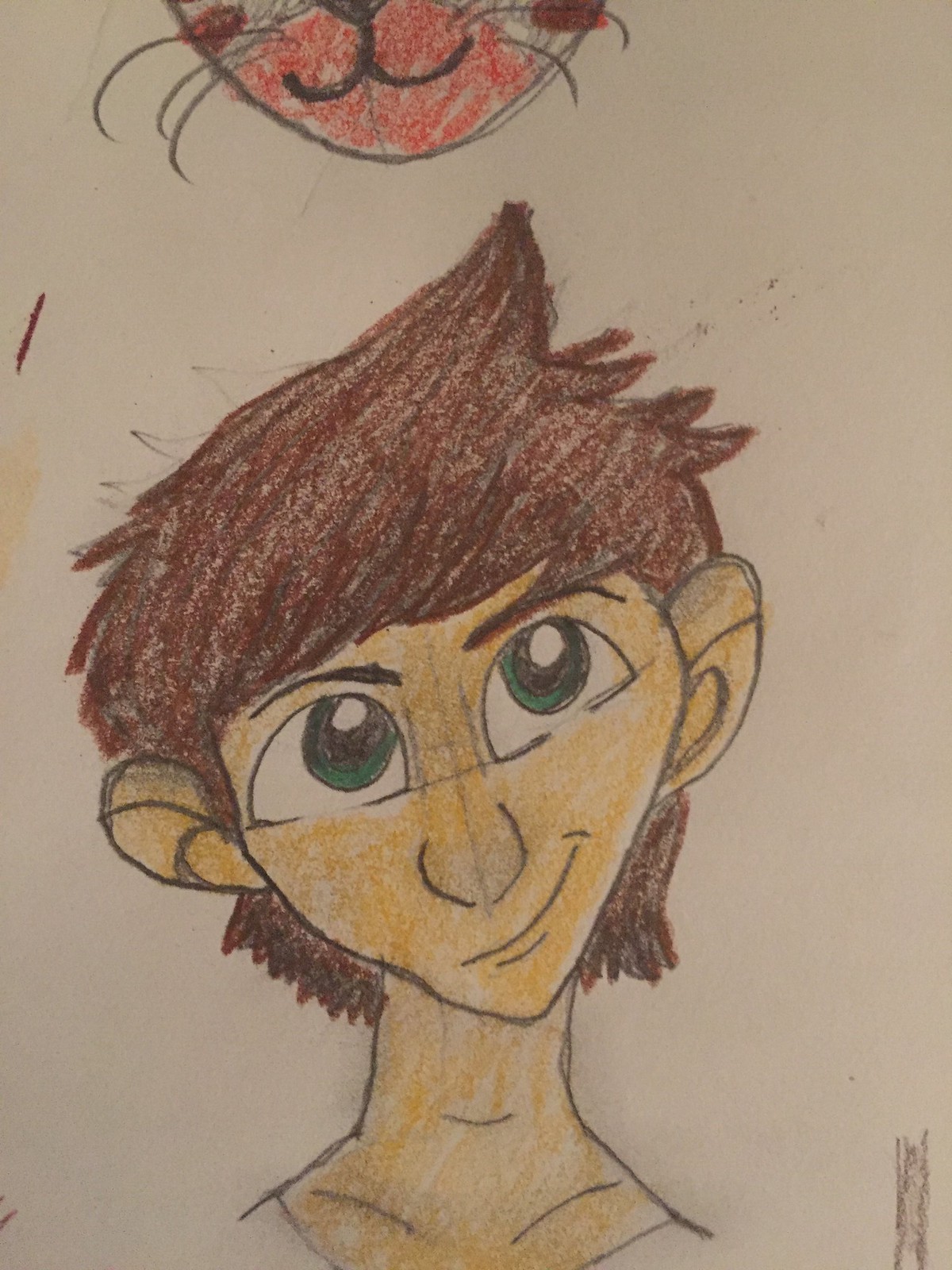The image is a highly detailed, hand-drawn colour illustration on a beige piece of paper, likely a digital scan due to its perfect appearance with no reflections. Dominating the bottom two-thirds of the image is a young man with reddish-brown hair that spikes upwards towards the right side. His hair has messy points sticking out and covers part of his dark eyebrows. He boasts striking turquoise green-blue eyes with large black irises, accented with white reflections at the two o'clock position. His face features a very pointed, triangular chin, and he offers a crooked smirk that tilts to the right side. The young man’s ears are quite large and protrude slightly, and his narrow neck shows some lines indicative of the clavicle area.

Above the young man, truncated at the top of the image, is the lower portion of an anthropomorphised cat's face. The cat’s mouth is defined by a double U shape descending from its central nose, with dark whiskers extending horizontally. The area around the mouth is roughly shaded in pink, not perfectly filled in, with additional soft gray fur around the mouth and cheeks. Colored pencils and crayons, possibly with some charcoal, have been used to create the illustration, resulting in an intricate and colorful piece of art.